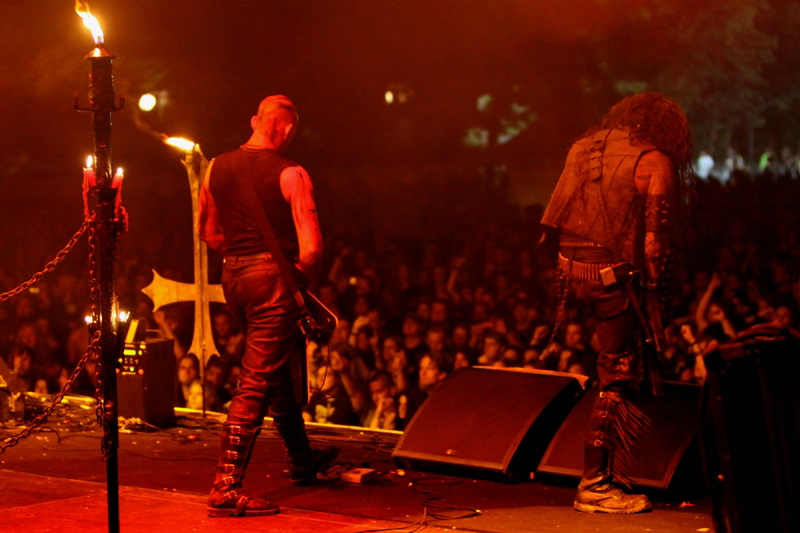The image portrays a high-energy rock concert, likely featuring the black metal band Gorgoroth, known for their intense stage presence and theatrical elements. Captured from behind the performers, the stage is bathed in a deep red glow, casting a dramatic atmosphere over the entire scene. Two male musicians, each wielding electric guitars, dominate the stage. The guitarist on the right, sporting long hair, is clad in leather pants, a sleeveless leather vest, and leather belts on his arm, while the one on the left wears leather pants, buckle-adorned boots, and a basic sleeveless black tank top. 

Flames flicker from wrought iron candelabras and an inverted flaming cross adds a provocative touch, emphasizing their punk-rock flair. Large speakers sit at the musicians' feet, with one guitarist propping his foot on a speaker, possibly engaging in a dynamic performance move, while the other might be adjusting a pedal. The dark, nighttime setting is animated by the vibrant energy of a massive crowd, whose raised hands and blurred, illuminated faces in the background reflect the fervent atmosphere of the performance.